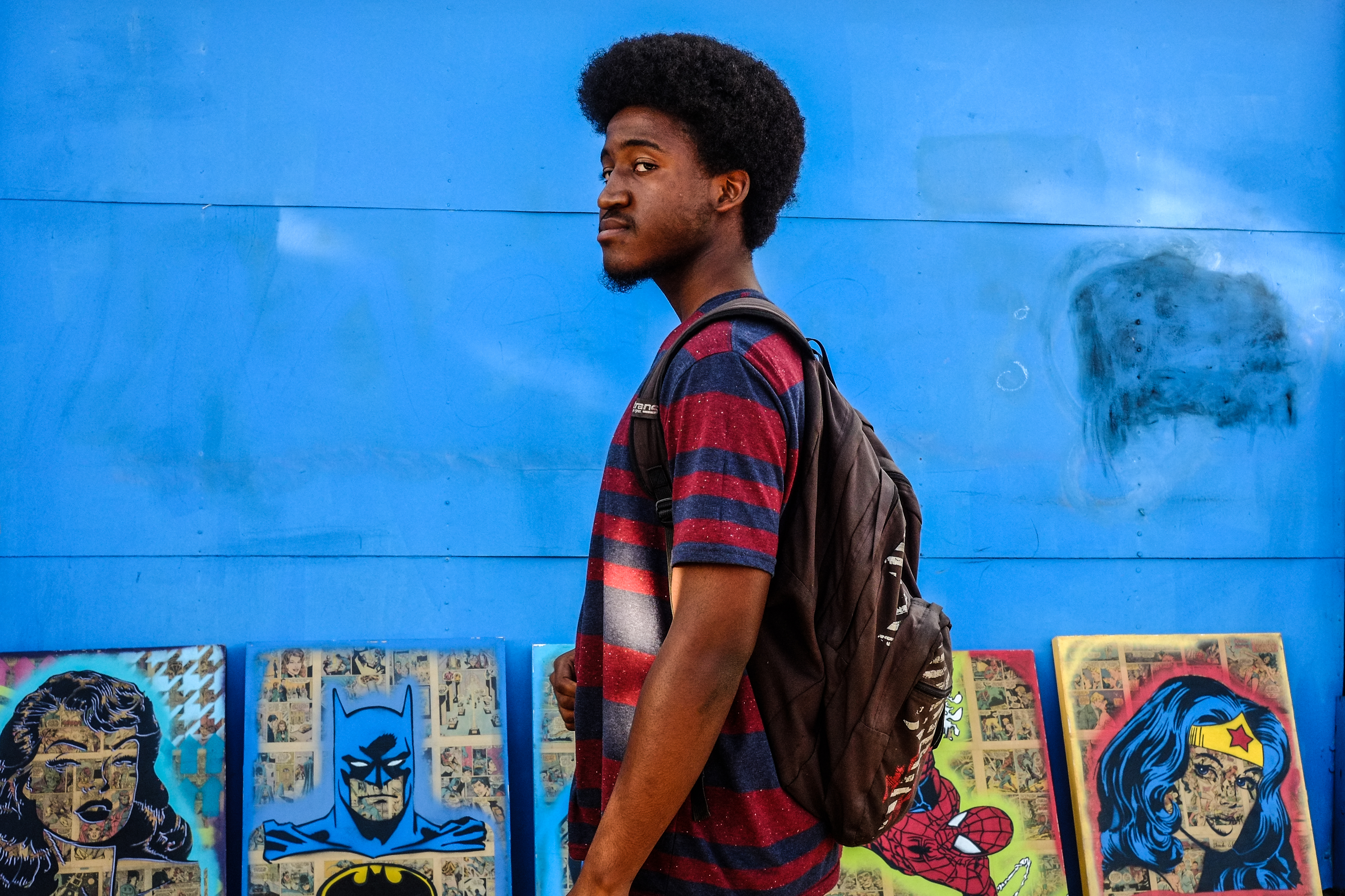The photograph features an African American young man, around 18 or 19 years old, who is possibly a student. He has a heavy afro at the front, shorter in the back, and sports some facial hair with a mustache and stubbles. His eyebrows are slightly raised, giving him a side-eye expression. Dressed in a red and blue horizontally striped t-shirt and carrying a brown backpack, he stands sideways against a brilliantly bright blue wall. The blue wall has rough, visible paint strokes and leans five vibrant, modern punk-style paintings featuring comic characters like Batman, Wonder Woman, and Spider-Man. These artworks prominently use a similar blue hue as the wall, suggesting a cohesive artistic theme; possibly indicating that he is the artist behind these striking pieces.